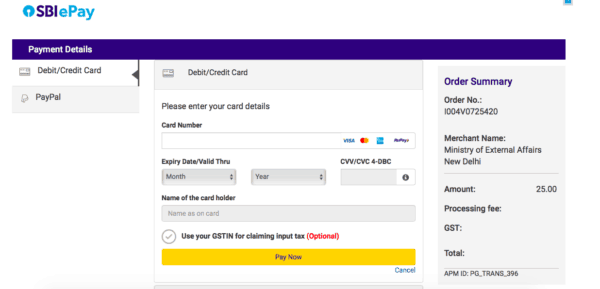The image displays an online payment page with a header that reads "SBI e-Pay." The "SBI" text is in purple while "e-Pay" is in blue. Below the header, a white "Payment Details" text is prominently displayed within a blue box. The payment form allows users to input their debit or credit card information, including fields for the card number, expiration date (selectable via month and year dropdown boxes), and CVV/CVC code. Accepted payment methods, depicted with icons, include Visa, MasterCard, PayPal, and an additional unspecified option.

There is a prompt to enter the cardholder's name exactly as it appears on the card. An optional field is available for entering a GSTIN for claiming input tax credits. The form includes a yellow "Pay Now" button for submitting the payment.

To the right of the form is an order summary detailing the order number, merchant name (Ministry of External Affairs, New Delhi), and the transaction amount of $25. There’s a section for processing fees, GST, and the total amount, although these fields are currently blank.

Overall, the colors used on the page distinguish different sections and action items: purple for "SBI," blue for "e-Pay" and the payment details background, and yellow for the "Pay Now" button. Additional instructional text identifies the CVV location on the card and provides guidance on its input.